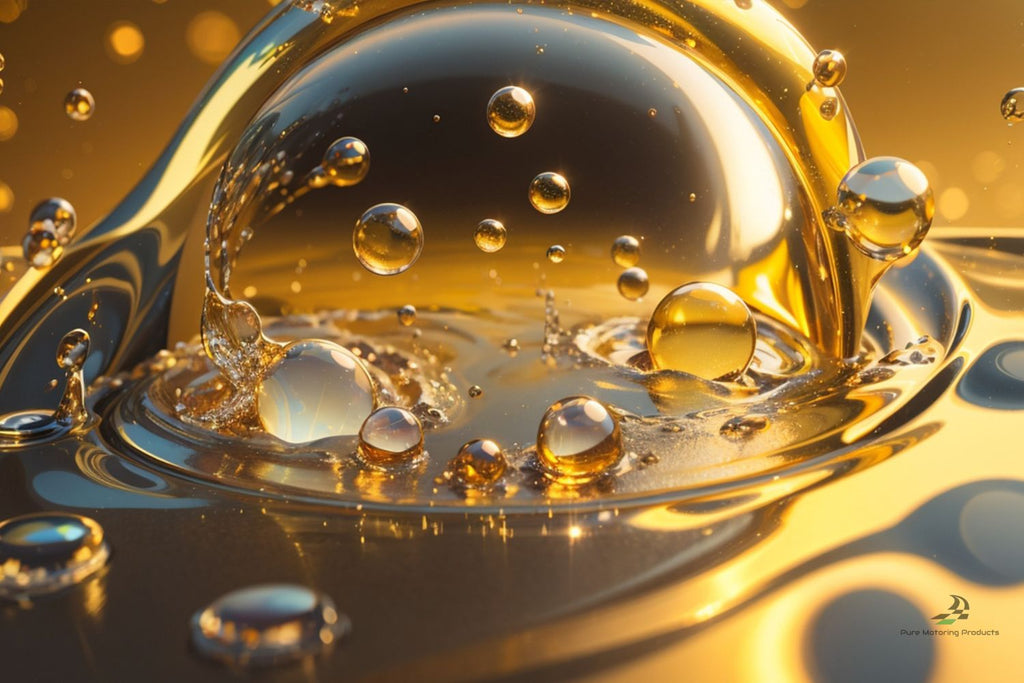The image appears to be a highly detailed, close-up shot, potentially rendered in 3D, capturing numerous water or oil bubbles suspended within a viscous, amber-gold liquid. Dominating the center is a large, circular bubble, which encapsulates several smaller bubbles within it, mimicking a nested, spherical arrangement. Surrounding this central bubble are various other bubbles of diverse sizes, creating a visually complex scene that is illuminated by a rich interplay of light, casting golden and yellow hues against a darker, almost black background. The scene evokes a sense of marbles floating in an otherworldly liquid or perhaps an artistic depiction akin to an astronaut's helmet immersed in fluid. At the bottom right corner, there is a distinct logo resembling a car with a checkered flag, accompanied by the text "Pure Motoring Products," suggesting an automotive association, possibly indicating that the liquid could be oil or gasoline.